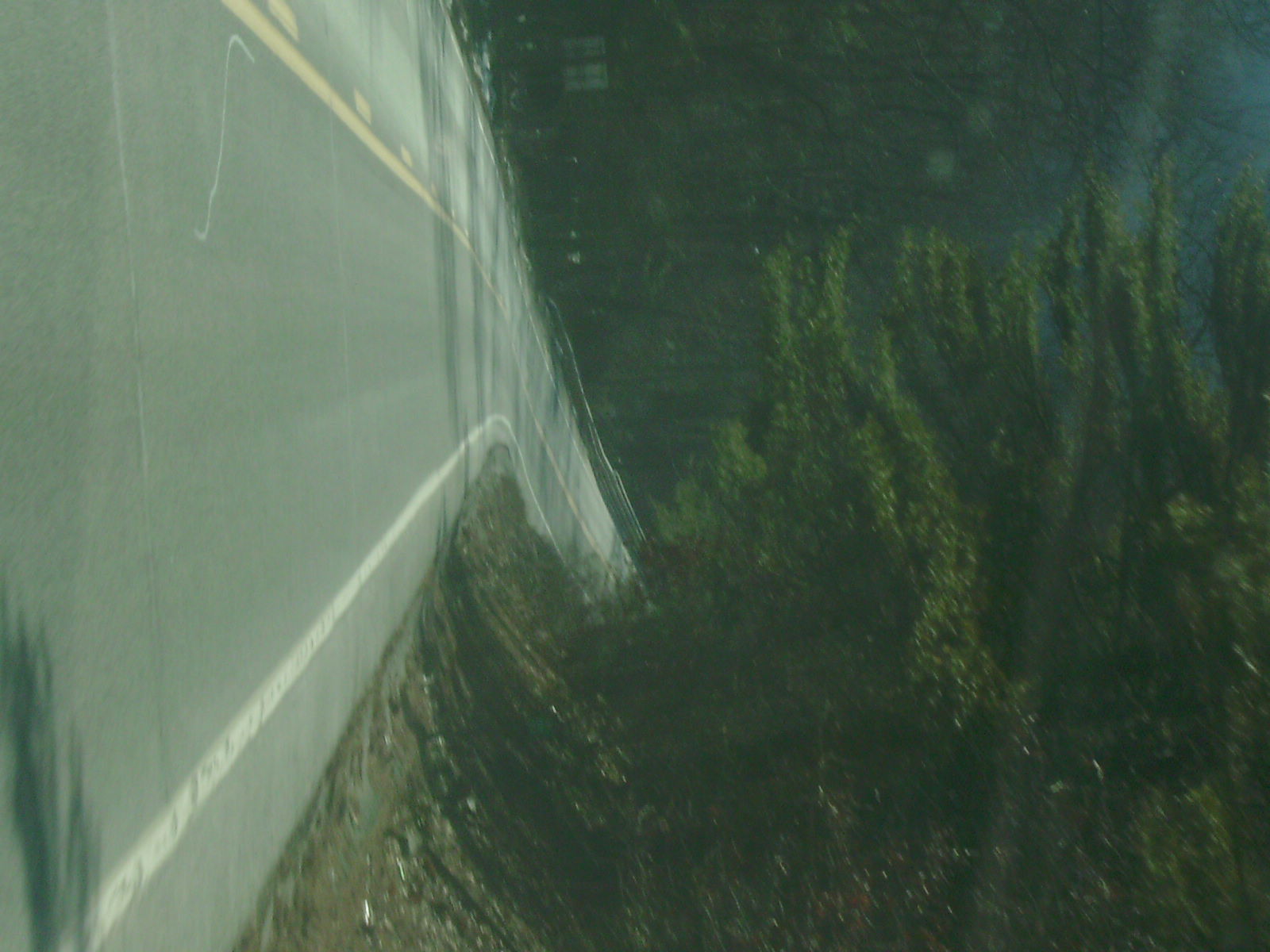The image depicts a first-person perspective taken from within a car, which has been rotated 90 degrees to the right. When viewed correctly, it shows a narrow, one-lane highway with a yellow line in the center separating the lanes. On the right edge of the road, a white shoulder line is visible, but the shoulder itself is small. The landscape surrounding the road features green vegetation and patches of dirt, suggesting the area is forested. Trees form a natural border on both sides, creating a tunnel-like effect. A reflective glare on the image, likely from a car's windshield, indicates it was taken through the front windshield of a moving vehicle. The light source, possibly the sun, appears to come from the top right, casting rays that enhance the greenish-blue tint of the scenery.